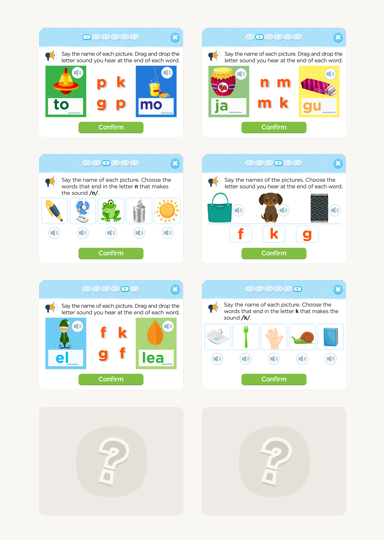In this screenshot, we observe a blurry interface showcasing children's educational cards, characterized by vivid and colorful prints. A prominent loudspeaker icon is visible in the top left corner, indicating an auditory cue for users to say the name of each picture. Below this, instructions prompt users to drag and drop the letter sound they hear at the end of each word.

On the left side, set within a green box, there is an image of a spinning top. On the right, a yellow mop and pail are displayed. The central part of the screenshot features four letters in bright orange text: "PKGP," repeated twice. Adjacent to this, another card depicts a colorful jar in the center, labeled with the letters "NMMK." Further to the right, another card showcases a pack of gum with yellow and purple stripes.

Beneath the main images lies a green confirmation box with "Confirm" written in white text. Additionally, in the lower center left, there are images of a pen, a fan, a frog, a can, and the Sun. Above these images, the instructions advise users to say the name of each picture and select the words that end with the letter "N," which makes the sound "N."